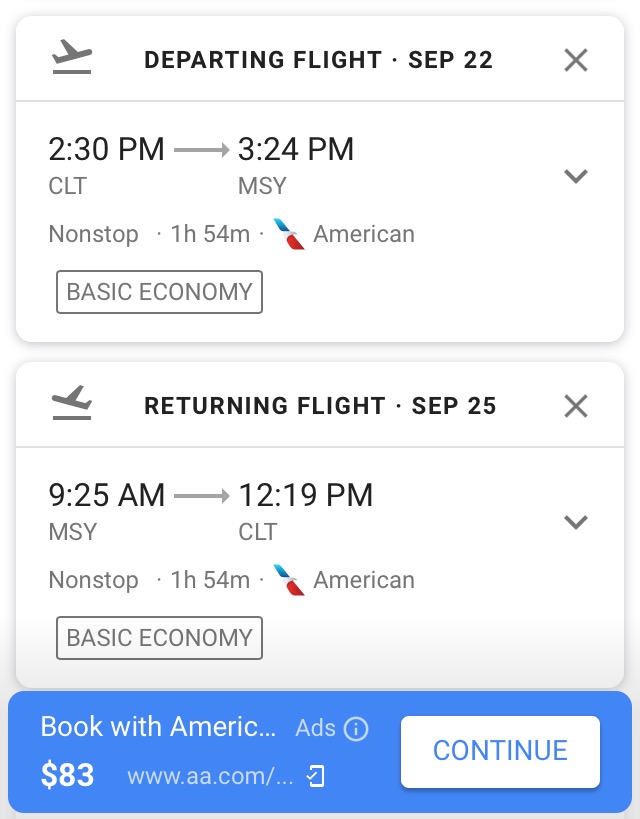This image is a screenshot of an American Airlines flight itinerary displayed on a smartphone. The website is laid out against a white background and features the American Airlines logo in several locations. 

At the top, the section is labeled "Departing Flight," scheduled for September 22nd. An airplane icon is shown next to this information. The flight details indicate a non-stop journey from 2:30 p.m. to 3:24 p.m., with a total duration of 1 hour and 54 minutes, under the "Basic Economy" fare class.

Below this, the "Returning Flight" information is presented for September 25th. The return flight is planned from 9:25 a.m. to 12:19 p.m., also non-stop, and similarly lasts 1 hour and 54 minutes in "Basic Economy."

At the bottom of the screen, the total price for these flights is listed as $83. A blue "Continue" button is prominently displayed, inviting the user to proceed with the booking.